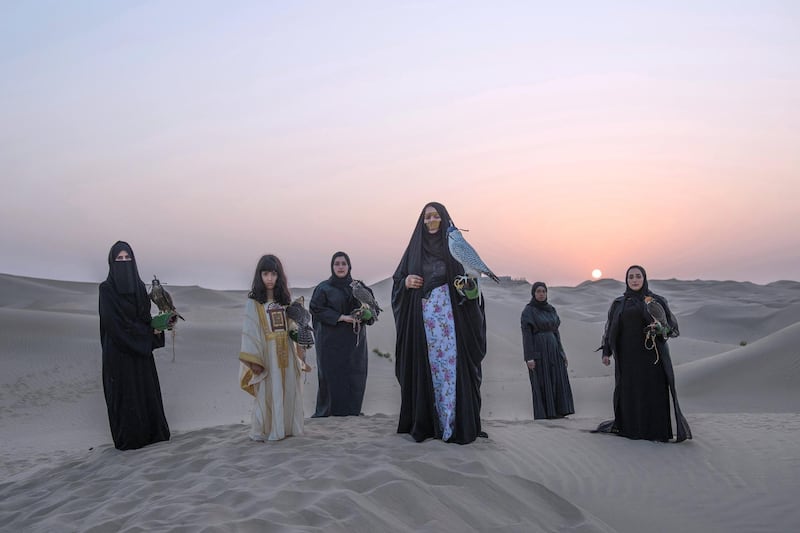This striking photograph captures six women standing on a small hill amidst the endless sand dunes of a desert, under an awe-inspiring sky either at sunset or sunrise. The sun, barely above the horizon on the right side of the image, bathes the scene in hues ranging from the deep reds and oranges near the horizon to the cool blues and purples higher in the sky. The women are arranged in a line, with one woman closest to the camera, and the others a couple of steps behind her, equidistant from one another.

All six women are part of a female falconry team, each holding a falcon with gloved hands, except one who is distinguished by her attire and posture. The woman nearest to the camera is adorned in a full black robe and a gold face covering, giving her an almost skeletal appearance due to the reflections and shadows. Three of the other women have their faces uncovered while wearing traditional Middle Eastern dress, only exposing their faces and nothing else. The intricate detailing of their garments against the stark desert landscape emphasizes the cultural richness of their attire. 

Among them, a younger girl stands out in a white and gold ornate robe, with long brunette hair flowing freely, unperturbed by the traditional headscarf restrictions that her companions observe. The seamless blend of cultural heritage, the natural beauty of the desert backdrop, and the unique presence of the falcons create a captivating and evocative image that speaks volumes about tradition, unity, and the untamed beauty of nature.